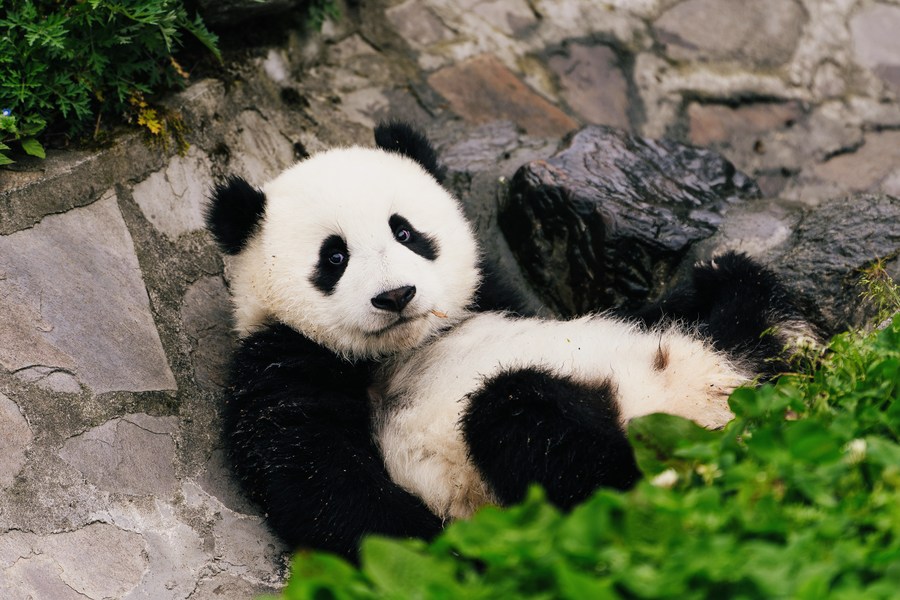In this outdoor daytime photograph, a panda bear is depicted reclining against a stone wall. The panda, with a white face, black ears, black patches around its eyes, black arms and legs, and a white belly that's slightly soiled, is looking directly at the camera with an almost human-like posture, exposing its belly. The stone wall behind it is comprised mainly of light and dark grey rocks, with the darker shade likely being the mortar. In the bottom right corner of the image, some green leaves are visible, adding a touch of nature to the scene. More green foliage is present in the top right corner, suggesting this setting could be an enclosure, possibly within a zoo. The panda's relaxed yet slightly attentive demeanor makes for an endearing and detailed capture.